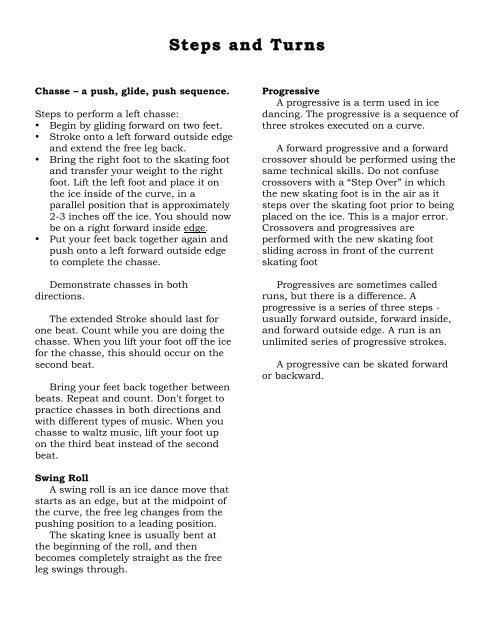The image depicts a page from an instructional manual, possibly a book for dance or ice skating techniques. This particular page focuses on detailed instructions for performing various dance moves, especially within the context of ice skating. 

It begins with the "chasse," a sequence comprising a push, glide, and push motion. The manual provides step-by-step directions: stroke the left foot forward on the outside edge, then bring the right foot to the standing foot and transfer your weight. An accompanying illustration or diagram demonstrates the correct position for the "chasse," aimed at guiding instructors on how to teach and properly execute the move.

The page also covers other dance maneuvers, such as the "swing roll," detailing the correct position and execution technique. Additionally, it includes a definition for "progressive," explaining it as a sequence of three strokes performed on a curve, specifically used in ice dancing.

Overall, the manual seems to be a comprehensive guide on dance and ice skating steps and turns, providing clear instructions and criteria for executing each move accurately.